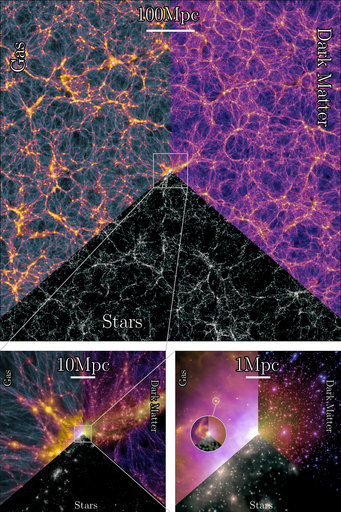This infographic consists of three panels arranged in a vertical sequence, each displaying a scientific comparison of different cosmic structures—dark matter, gas, and stars—through various telescope zoom levels. In each panel, three distinct sections are present: the top left segment shows 'Gas' represented by an orange and black pattern, the top right segment shows 'Dark Matter' depicted with purple and white lines, and the bottom triangle shows 'Stars' characterized by black with white smoke-like lines.

The topmost panel is labeled "100 MPC," with the dark matter section resembling a purple plasma and the gas appearing as volcanic black gas. The middle panel, marked "10 MPC," shows the same segments but introduces golden glowing light streaks into the dark matter and gas sections. The bottom panel, labeled "1 MPC," intensifies this effect, presenting brighter and more prominent light bursts across all three segments. Each panel reinforces the comparison with vibrant colors, including purples, yellows, pinks, and blacks. At the bottom of every panel, the word "Stars" appears in the triangular section. 

Overall, this detailed infographic uses varying zoom levels—100 MPC, 10 MPC, and 1 MPC—to illustrate distinct visual characteristics of dark matter, gas, and stars in space.